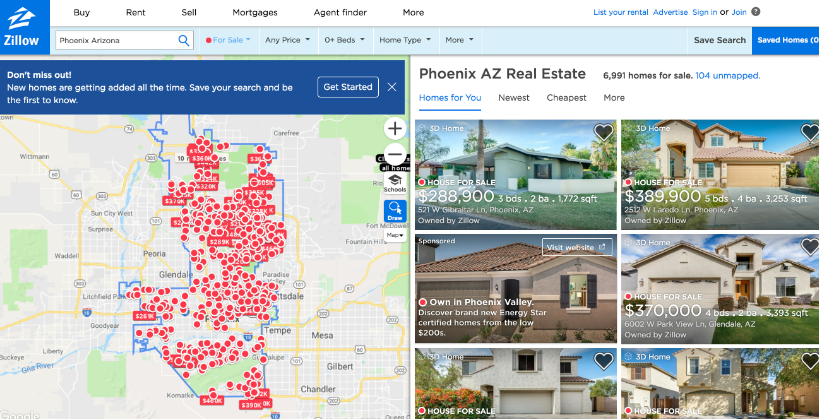This is a detailed screenshot of the Zillow website, which is a popular real estate platform. The distinct Zillow logo is prominently displayed in the top left corner. At the very top of the page, a white header banner allows users to navigate through various options such as "Buy," "Rent," "Sell," "Mortgage," "Agent Finder," and "More." Immediately below this header, there's a compact search bar flanked by filters labeled "For Sale," "Any Price," "Number of Beds," "Home Type," and "More."

On the left side of the webpage, a detailed map displays the Phoenix area in Arizona, with several red dots marking properties that are either for sale or rent. This includes the central city and its surrounding suburbs. On the right side of the webpage, there's a panel featuring images and details of homes available in the Phoenix area. The top of this panel reads "Phoenix, Arizona Real Estate" and indicates that approximately 7,000 homes are currently for sale. Displayed within the panel are six images of various homes, showcasing a range of property types. The prices of these homes vary, with listings starting at $280,900 and going up to $3,370,000.